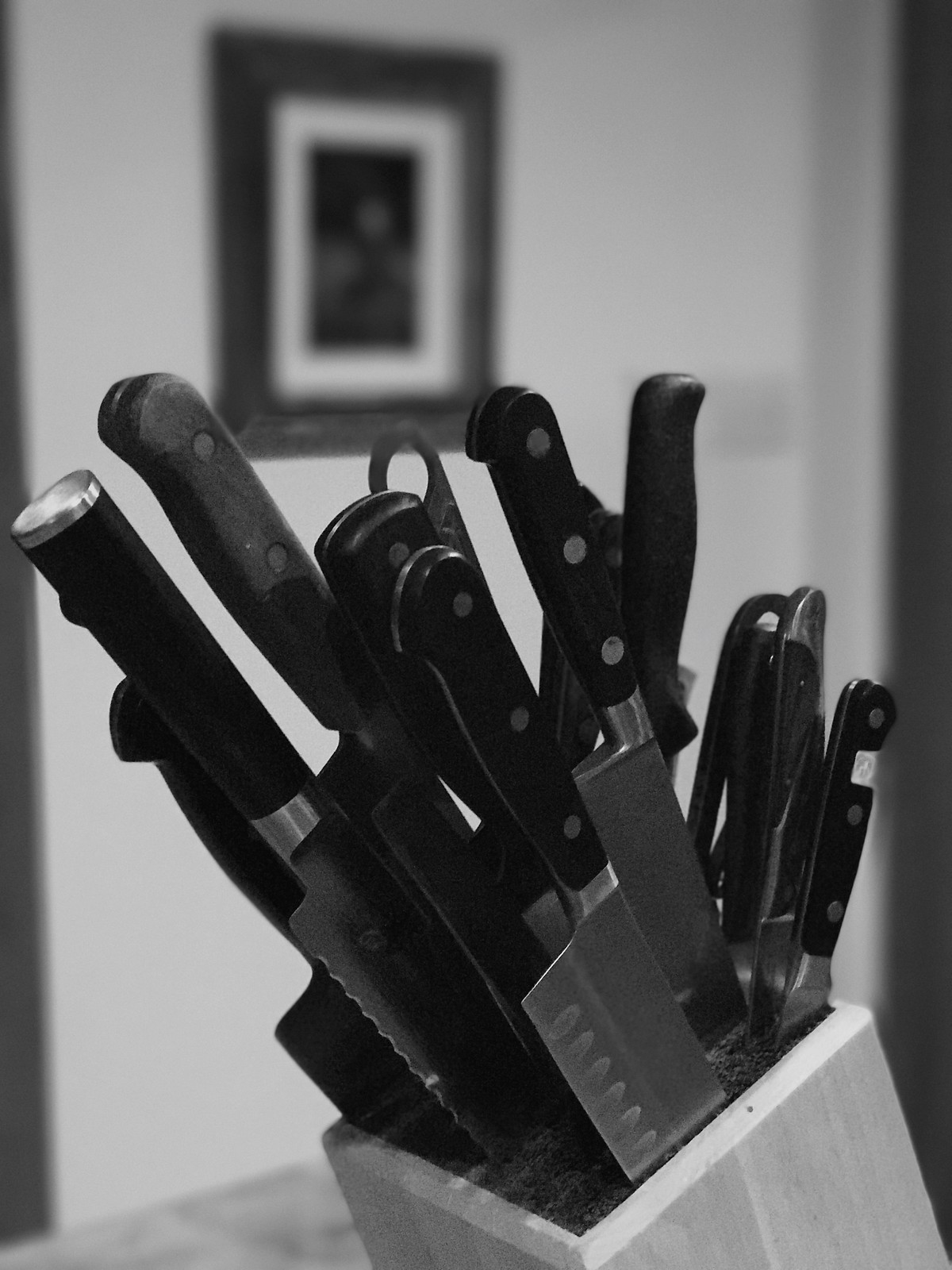This black-and-white photograph, taken in portrait orientation, features a close-up view of a kitchen knife block. The wooden knife block is partially cut off, showing primarily the handles of the knives extending upward. The handles are black with two to three rivets, and they exhibit varying shapes, including rounded and flatter designs. Some of the stainless steel blades are visible, protruding from the overcrowded block, which even contains a pair of scissors, indicating that the set includes different types of knives such as paring, butcher, carving, and bread knives.

The background, though blurred, reveals a light-colored wall with a prominently framed artwork or photograph. The frame is dark, encasing a lighter border with a darker image at its center, adding a touch of decor to what appears to be a kitchen countertop scene. This focus on the sharp, detailed knives against the softer, out-of-focus background creates a striking depth of field in the monochromatic image.